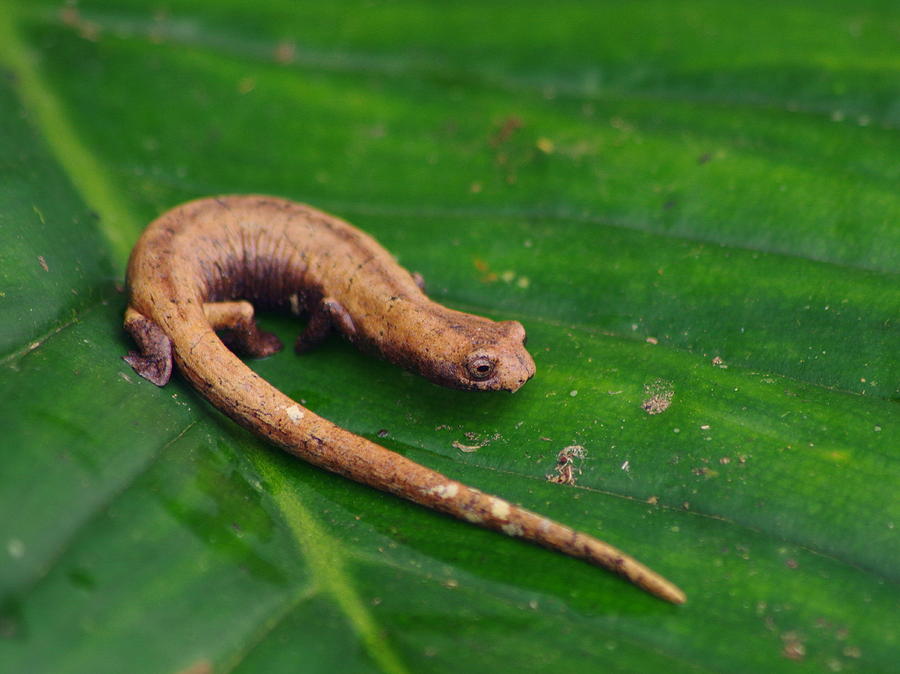This close-up image showcases a small brownish-beige reptile, likely a newt or salamander, perched atop a dark green leaf. The detailed shot captures the creature's bulging eyes and four legs; two positioned behind its neck and head, and two placed after the bend of its body. The newt's form is gracefully curved in a U-shape, facing the bottom right side of the image, with its tail aligned parallel to the orientation of its head and body curve. The leaf beneath is speckled with subtle brown spots, possibly remnants of raindrops or dust, giving it a slightly cloudy texture. Prominent veins run through the leaf, adding depth to the vibrant green backdrop against which the small creature is vividly highlighted.